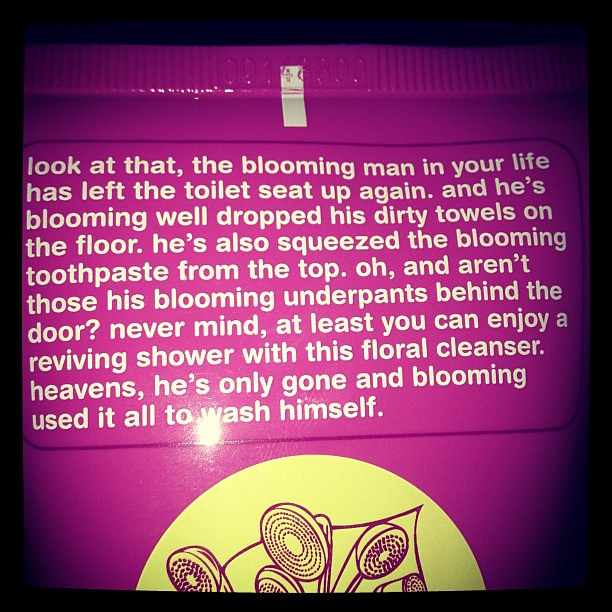The image illustrates a nearly square, purple sealed package intended for use in the shower, primarily targeting women. Dominating the center of the image is the product, which features a pull-tab similar to those found on grocery items. The bottom portion of the package, cut off about halfway, includes a prominent yellow half-circle adorned with illustrations of shower heads in purple. Conspicuously, a large white font displays text with an Australian twist, humorously recounting various bathroom misdeeds by a man—such as leaving the toilet seat up, abandoning dirty towels, and improperly squeezing the toothpaste. The message humorously acknowledges these annoyances and sarcastically comforts the reader by suggesting they could enjoy the reviving floral cleanser—only to reveal that the blooming man has already used it all up. The overall tone is light-hearted and comedic.